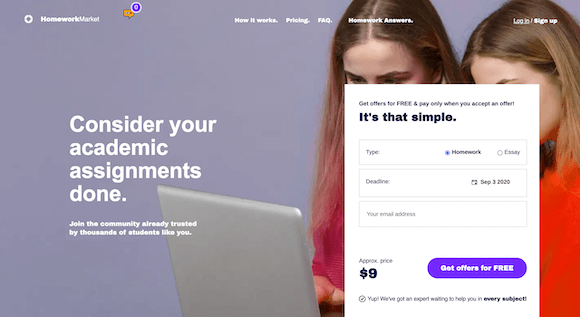**Website Homepage Screenshot: Detailed Description**

The image is a screenshot of the homepage of a website named "Homework Market," as indicated by the name displayed prominently at the top-left corner. The central focus of the page features a bold statement: "Consider your academic assignments done. Join the community already trusted by thousands of students like you." This message encourages users to become part of a large, established network.

To the right of this central message, there is a white, interactive box. At the top of this box, a headline assures users: "Get offers for free and pay only when you accept an offer." Below this, the simple process is emphasized with the tagline: "It's that simple."

The interactive box includes specific fields to fill out:
1. A dropdown menu or selection box labeled "Type," where users can choose between options such as "homework" or "essay." The "homework" option is currently highlighted.
2. A "Deadline" section, likely where users can specify the due date for their assignment.
3. A text box labeled "Your email address" where users must input their contact information.
4. An estimated cost section reads "Approximate price $9" located on the left side.
5. A prompt for action, "Get offers for free," is positioned on the right side of the box, enticing users to move forward with the service.

This detailed structure aids users in understanding the process of obtaining help with their academic work, emphasizing ease of use and community trust.